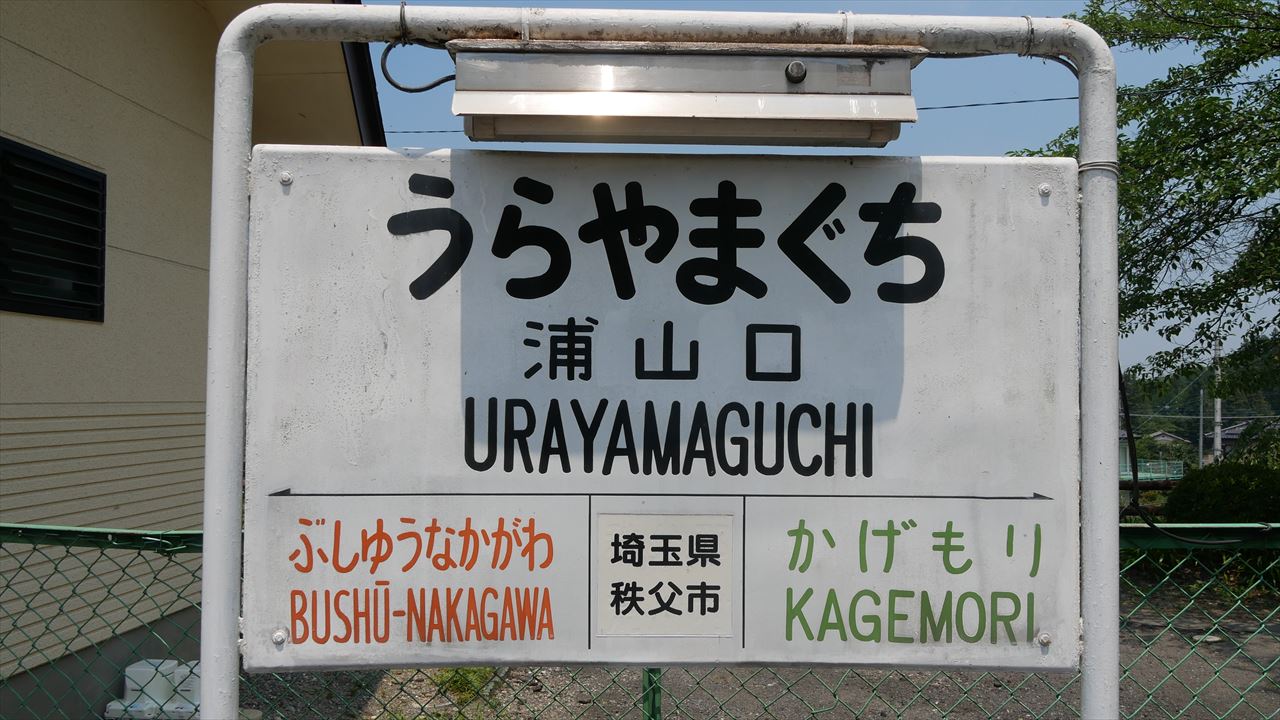A photograph captures a white metal sign framed between two vertical metal poles that rise from the bottom and stretch out of the photo's top edge, forming a rectangular pipe outline. The sign, which appears to be made of a solid white metal, is suspended between the poles, with a metallic structure—possibly a light—situated just above it.

The sign prominently displays black bolded Japanese characters at the top, followed by the romanized text "URAYAMAGUCHI" in black letters. Below this, the sign is divided into three sections with a horizontal black line separating them from the upper text. The left section contains red Japanese text, the middle section features black Japanese characters, and the right section has green Japanese text.

Surrounding the sign, the backdrop reveals more details: to the left, there's a tan building with black window shutters and white wall elements, along with some white boxes at the ground level near the bottom left. A green-painted chain-link fence runs behind the sign, stretching from left to right, with a dirt ground visible just beyond it. On the right side of the photograph, a few trees and a distant hill can be seen.